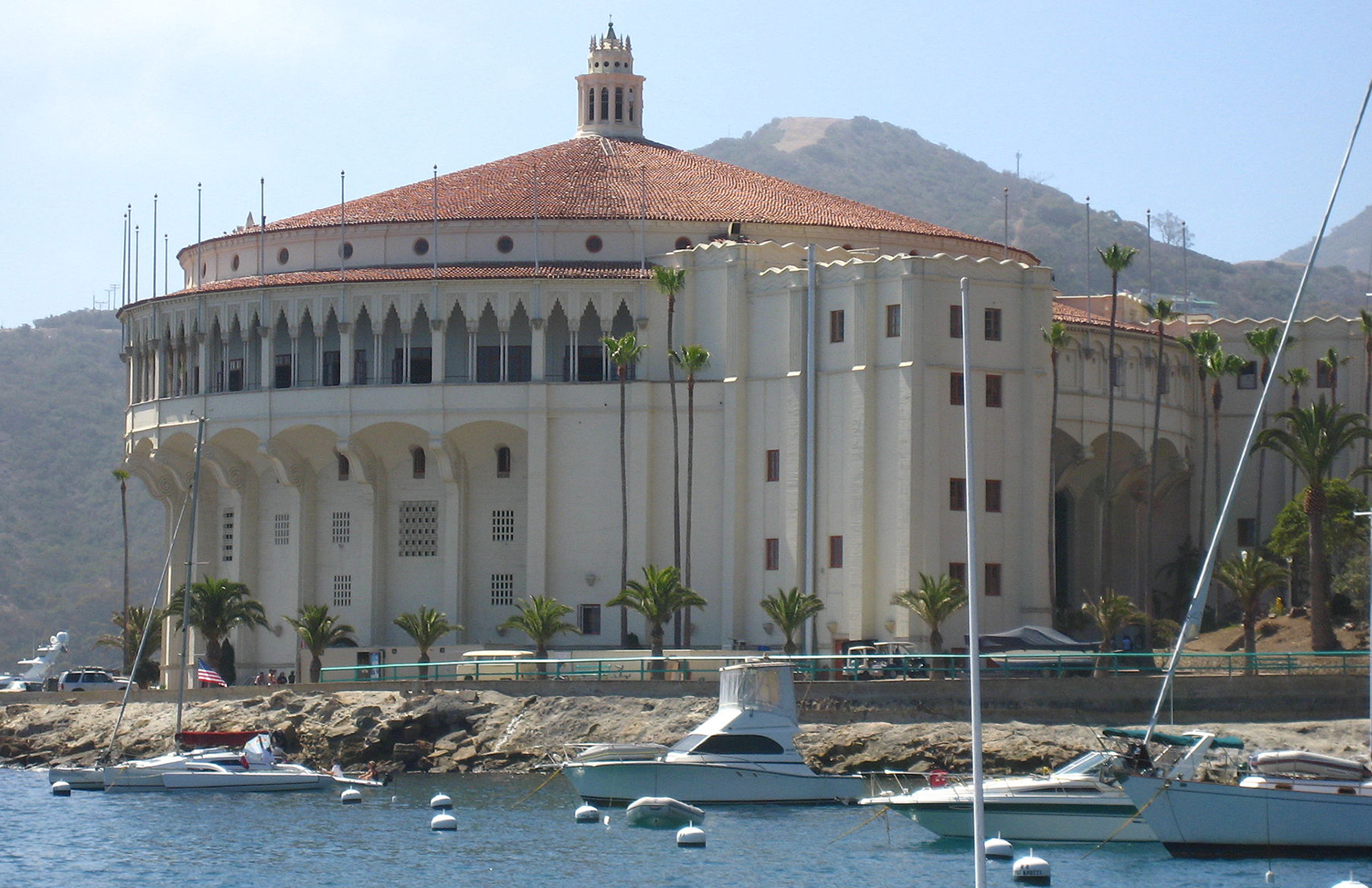The image shows a large, palatial tan building with a distinctive round architecture and a terracotta orange, shingled roof crowned by a widow's peak. The building's façade features many columns and numerous windows, some of which are not typical for residential use as they are not designed for visibility. Metal poles are visible, suggesting either ongoing construction or a specific functional purpose, such as flag holders. The upper floors of the building include deck areas framed by columns, enhancing its grand appearance.

Surrounding the building are lush palm trees and part of the yard is enclosed by fencing. In the foreground, a body of water hosts several medium-sized white boats, with buoys scattered around them. The boats are either docked or positioned from side views, with one visible near a dock to the left. Behind the building, a hill or mountainous area with vegetation provides a scenic backdrop. The day is beautifully sunny, with clear skies and a few clouds, accentuating the grandeur and elegance of the property.